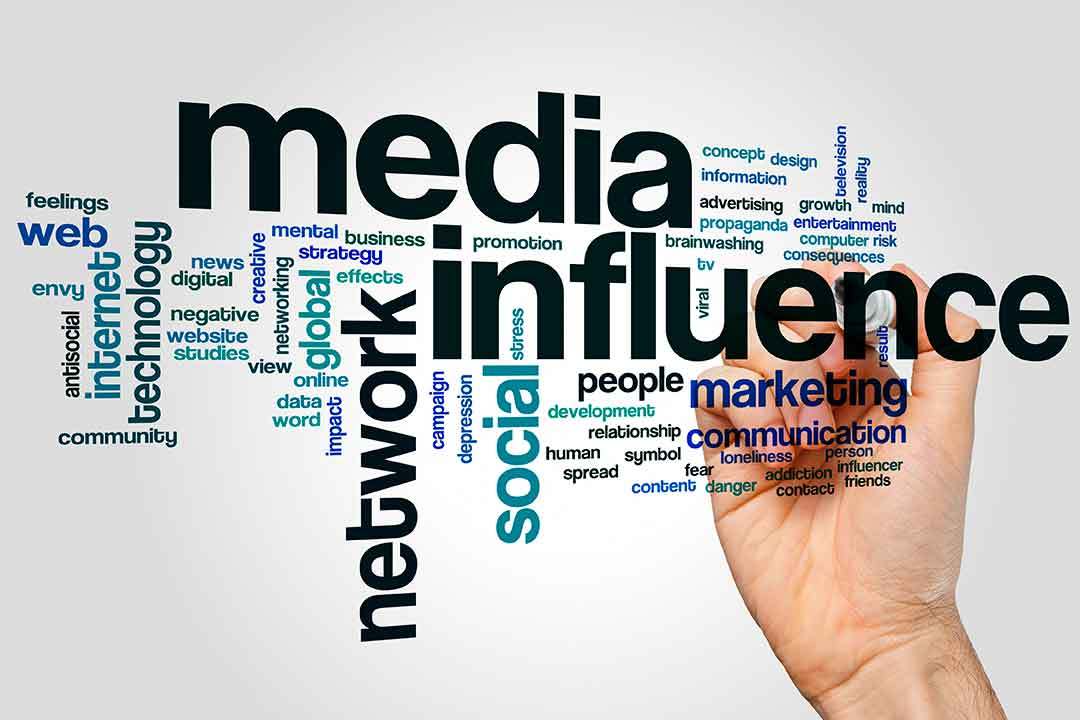The image features a "wordle"-style brainstorm depicting a complex network of words in varying sizes and colors, with the most prominent words being "media" and "influence" in large black letters. Surrounding these central terms, a multitude of smaller words—such as "network," "social," "feelings," "web," "envy," "antisocial," "community," "internet," "technology," "news," "digital," "negative," and "website"—are scattered in green, blue, purple, and black fonts. Additional words like "studies," "creative," "networking," "view," "mental," "business," "strategy," "global," "effects," "online," "data," "impact," "promotion," "campaign," "depression," "stress," "concept," "design," "information," "advertising," "propaganda," "brainwashing," and "TV" also appear. Toward the right side of the image, a hand is holding a marker, seemingly responsible for drawing the words. The background transitions from white in the center to a light gray gradient, providing a neutral canvas for the colorful and varied typography. The image effectively conveys themes of media, influence, and network connections, highlighting both positive and negative aspects.